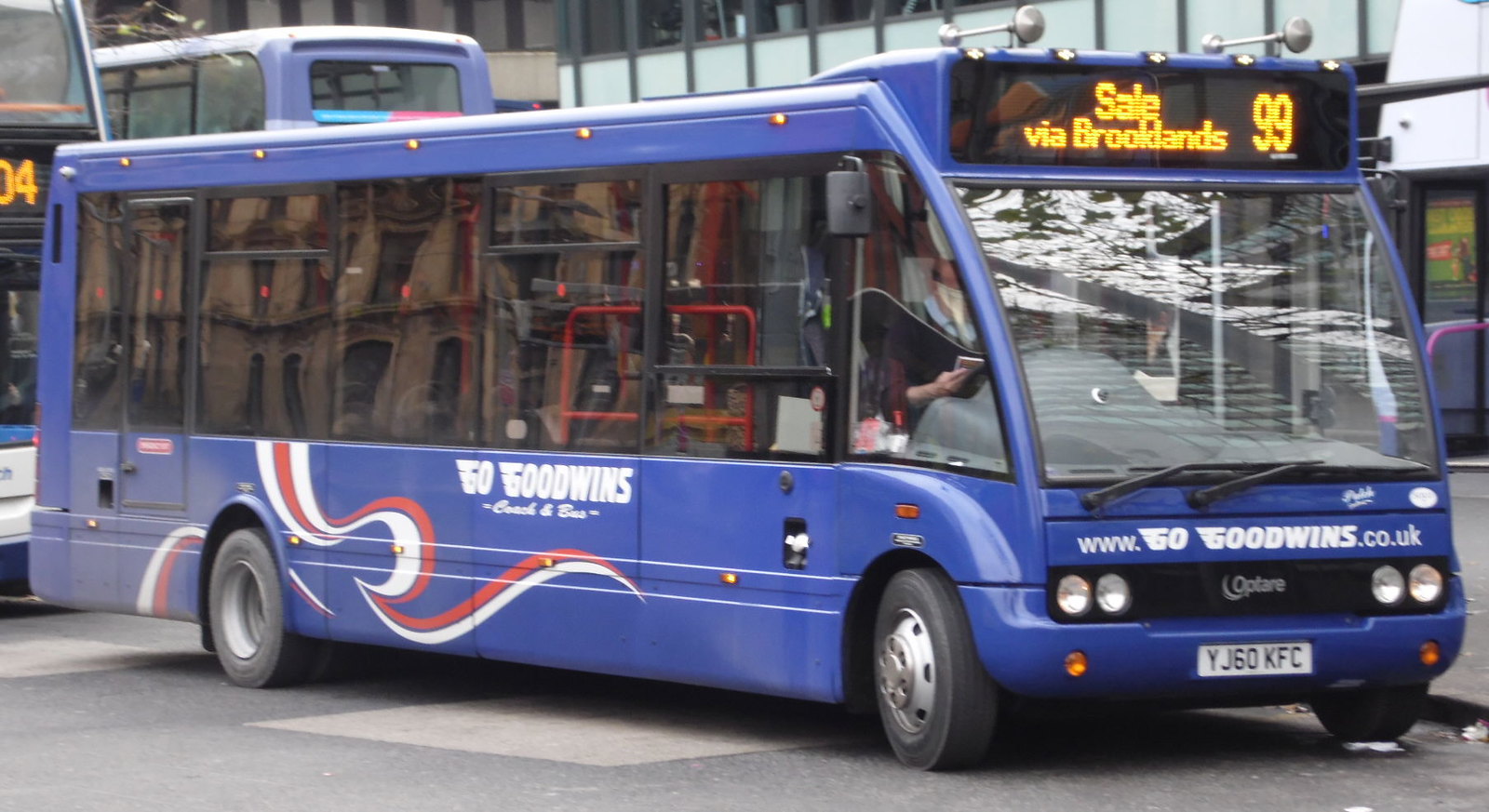The image is a detailed side view of a public city bus in a striking shade of blue, stretching across most of the frame. The bus features large, dark-colored windows set in black frames along its side and front, emphasizing its sleek design. The expansive windshield at the front is complemented by the bus's black grill, which bears the silver brand name "Optane." Just below the windshield, white text displays the website "www.gogoodwins.co.uk," and along the side, "Go Goodwins" is also prominently written in white. The bus sports a white European-style license plate with the characters "YJ60KFC" in black. A notable feature is the LED screen on the front, which reads "Sail Via Brooklands 99" in golden letters and numbers. The bus has double headlights, two on each side. The driver, partially visible, appears to be holding a pamphlet or a book, though their face is not clear. In the background, one can glimpse other buses and city buildings, indicating a busy urban setting.